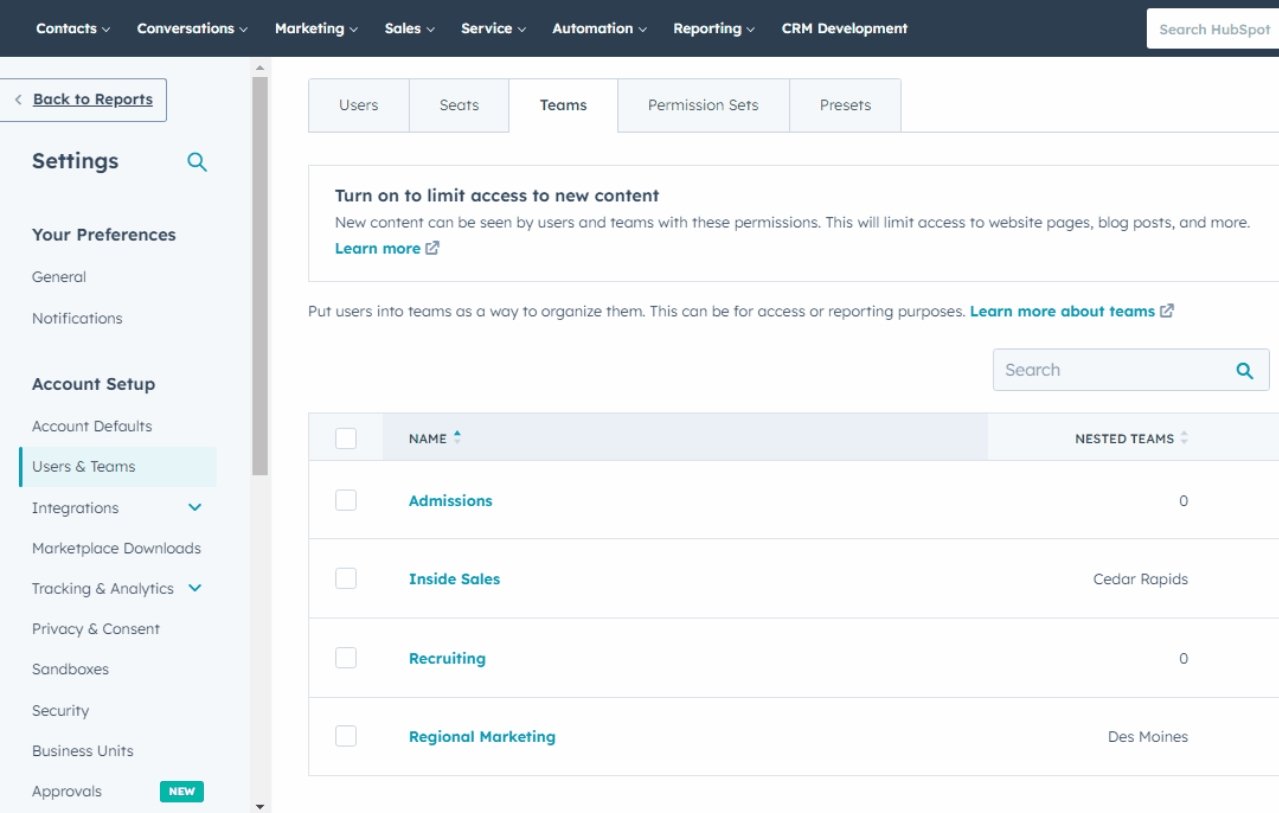The image appears to be a screenshot of a section within the HubSpot website interface. The browser elements like the URL bar are not visible, suggesting a focus purely on the website's content.

At the top of the interface, a black horizontal banner spans across, containing several tabs in white text. These tabs include "Contacts," "Conversations," "Marketing," "Sales," "Service," "Automation," "Reporting," and "CRM Development." Each of these tabs, except for "CRM Development," features a drop-down arrow indicating further sub-options. On the far right of this banner lies a search bar labeled "search HubSpot," reinforcing that the website in focus is likely HubSpot.

Beneath this dark banner, there's a light blue vertical sidebar running along the left-hand side. The first option in this sidebar is "Back to reports," which likely allows users to navigate to a previous page. Below this, in bold, is "Settings," followed by sections for "Preferences" (including subsections for "General" and "Notifications") and "Account Setup." The user is currently within the "Users and Teams" category, which is currently highlighted in this sidebar.

Adjacent to the left sidebar, the main content area for "Users and Teams" is displayed. This section is divided into five tabs at the top: "Users," "Seats," "Teams," "Permission Sets," and "Presets," with the current focus on the "Teams" tab. Below these tabs, a banner informs users that they can "turn on to limit access to new content." Further down, a searchable list of teams is presented, with teams such as "Admissions," "Inside Sales," "Recruiting," and "Regional Marketing" listed alongside checkboxes and corresponding value columns for each team. The bottom of this section features a gray banner with additional selectable options.